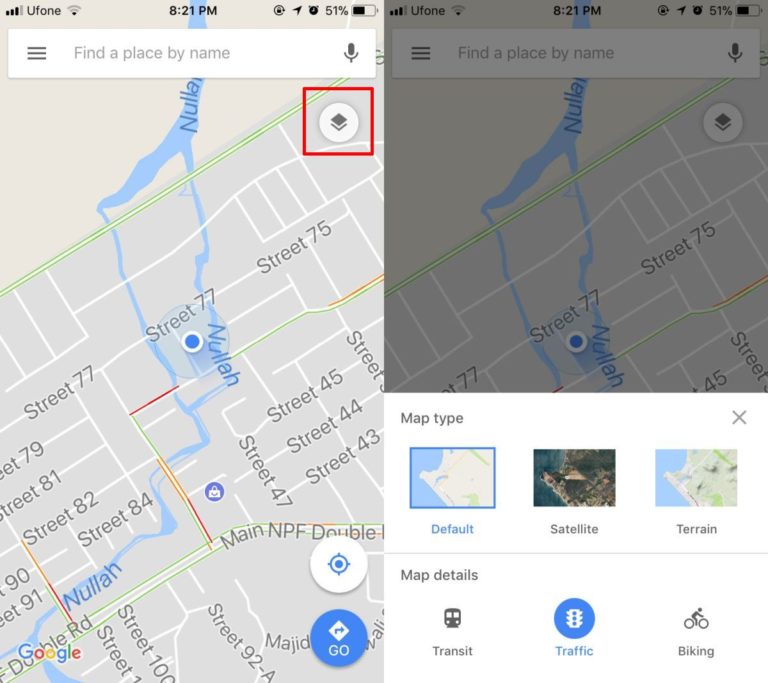In the image, two maps are displayed side-by-side. The left map prominently showcases "Street 77, Nullah," marked by a blue dot, indicating the user's current location. Above the map interface, "Uphone" is displayed, along with icons showing cellular signal, Wi-Fi signal, the time (8:21 p.m.), a battery level of 51%, and a search bar labeled "Find a place by name." At the bottom right of this map, there is the Google emblem.

This map interface also includes two circles at the lower right corner: a white circle with a blue bullseye icon and a blue circle with the word "GO" and a right-pointing arrow.

To the right of this main map, a smaller, darker, more focused map is shown. Below this smaller map, the interface includes options for various map types and details. The "Map Type" section features a blue-outlined square labeled "Default" in blue, a square labeled "Satellite" in gray, and another labeled "Terrain" in gray. These options allow the user to switch between different views of the map.

Below the map type options, the "Map Details" section presents various toggles: "Transit" with a bus emblem, "Traffic" indicated in blue with a traffic light icon, and "Biking" in gray with an icon of a cyclist.

Overall, the image showcases a comprehensive view of the Google Maps interface, with detailed information about map types, additional map details, and the user's current location.